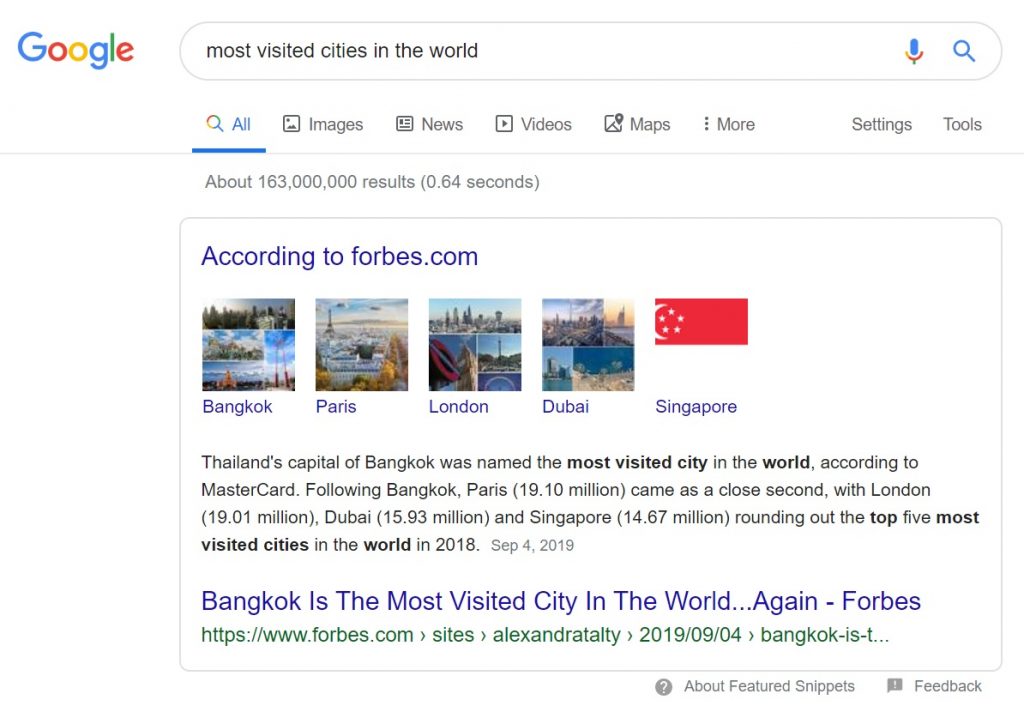The image depicts a Google search results page with the iconic Google logo at the top, featuring its recognizable colors of blue, red, yellow, and green. In the search box are the words "most visited cities in the world," accompanied by a colorful microphone icon and a blue search button. Just below the search bar, there are various filter options such as 'All,' 'Images,' 'News,' 'Videos,' 'Maps,' and 'More,' alongside 'Settings' and 'Tools' options.

At the top of the search results, a snippet from Forbes.com appears, listing the world's most visited cities. There are individual images of each city, starting with Bangkok, which showcases an expansive view of the cityscape. Paris is next, highlighted by an image featuring the iconic Eiffel Tower and other landmarks. London follows, represented by images including Big Ben. Dubai is also listed, accompanied by various illustrations of its skyline. Lastly, Singapore is featured, depicted alongside the country's red and white flag.

Beneath these images, a text box provides detailed information, stating: "Thailand's capital of Bangkok was named the most visited city in the world according to MasterCard. Following Bangkok, Paris, 19.10 million, came as a close second. London, 19.1 million, Dubai, 15.93 million, and Singapore, 14.67 million, rounding out the top five most visited cities in the world in 2018." This entry is dated September 4, 2019, and is sourced from an article titled "Bangkok is the most visited city in the world, again," by Forbes magazine. The web page features a predominantly white background with black text, providing a clean and straightforward layout for easy reading.